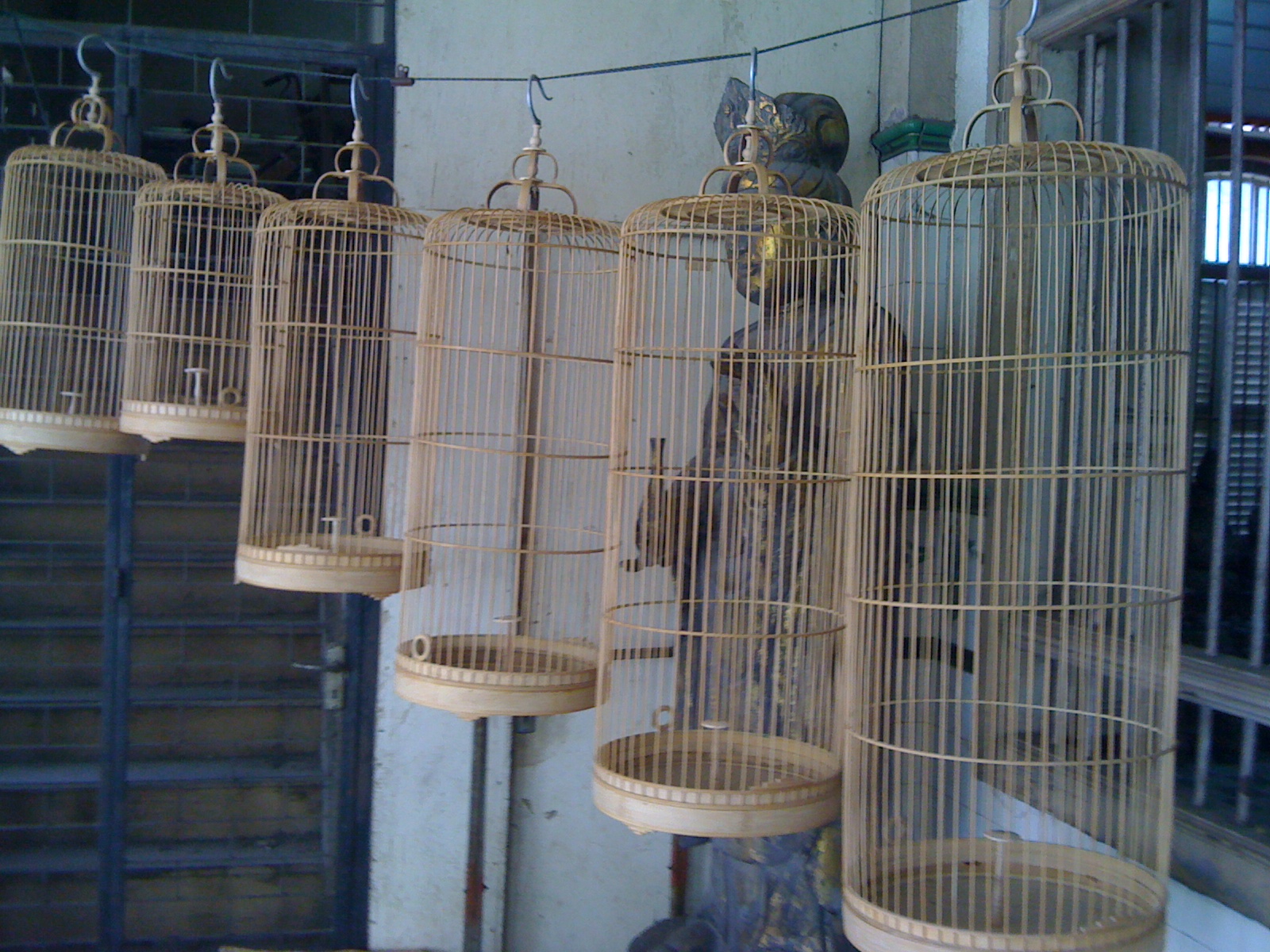An angled photograph showcases a line of six intricately designed white bird cages, each suspended from a thin wire by silver hooks. Arranged in descending order of size from right to left, the tallest cage on the far right gradually gives way to smaller cages, culminating in the shortest one towards the left. All the cages share the same elegant, elongated design and metallic texture, yet they vary in height. Behind the cages, set against a stucco-like white building exterior with barred windows and a black metal gate, stands a tall wooden statue of a Chinese character with one hand raised. The clean, birdless cages and the serene statue collectively evoke a sense of tranquility and meticulous artistry.